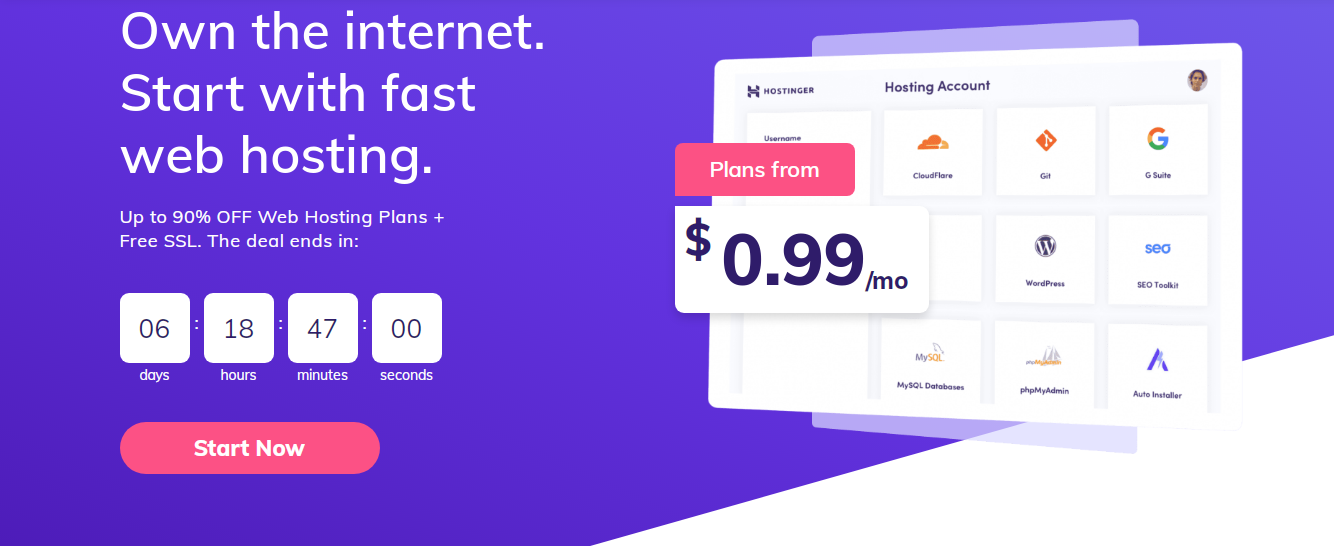The image features a promotional graphic set against a vibrant purple background. At the top, text highlights an internet deal starting with fast web hosting services. The promotion offers up to 90% off on web hosting plans along with free SSL certificates. A countdown clock indicates that the deal ends in six days, 18 hours, 47 minutes, and 00 seconds. 

Central to the image is a red oval button with the text "Start Now" written in white. Below this, there is a screenshot of a computer display. The screenshot itself is within a white rectangular frame and shows a grid of app icons or logos, suggesting a user interface. In the top right corner of this screenshot, a profile picture is visible next to text that says "Hosting Account." Beneath this, a red rectangle with white text promotes plans starting from a certain price, which is shown in a white rectangular box with a purple "$.99/MO" highlighted.

This detailed caption thoroughly describes the visual elements and promotional content of the image.